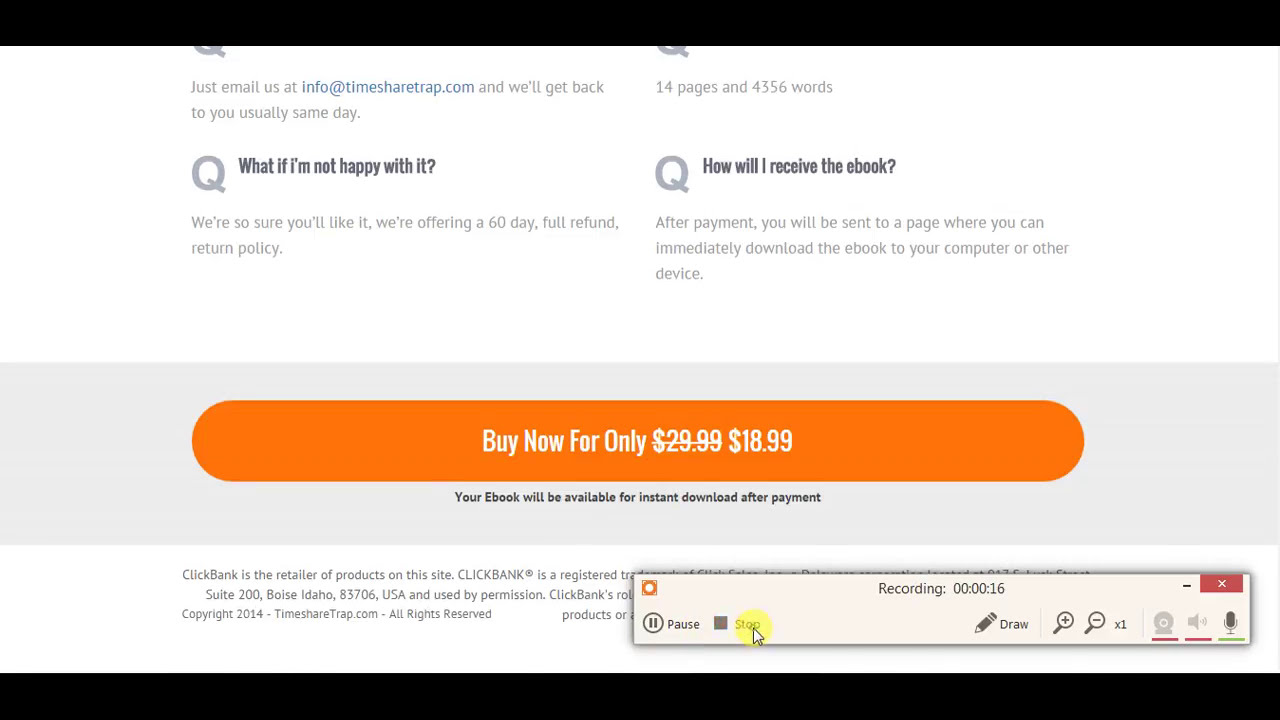This image is a screenshot capturing a website, likely an FAQ section, displaying details about purchasing an ebook. Key elements include the text “Just email us at info [at] timesharetrap.com and we'll get back to you usually the same day,” with the email address hyperlinked and in blue font. There are several questions with corresponding answers: One question asks, “What if I'm not happy with it?” and the answer guarantees a 60-day full refund return policy. Another question related to the ebook's format reveals it consists of 14 pages and 4,356 words. For delivery, the question “How will I receive the ebook?” is answered with “After payment, you will be sent to a page where you can immediately download the ebook to your computer or other device.” Prominently featured in the lower third of the webpage is a wide, orange button with the text “Buy now for only $18.99,” with an original price of $29.99 crossed out, indicating a discount. Below it, a message confirms the ebook will be available for instant download post-purchase. The screenshot also captures a recording utility window in the bottom right corner, containing tools for pause, stop, zoom, and audio adjustments, suggesting that the screen was being recorded at the time.